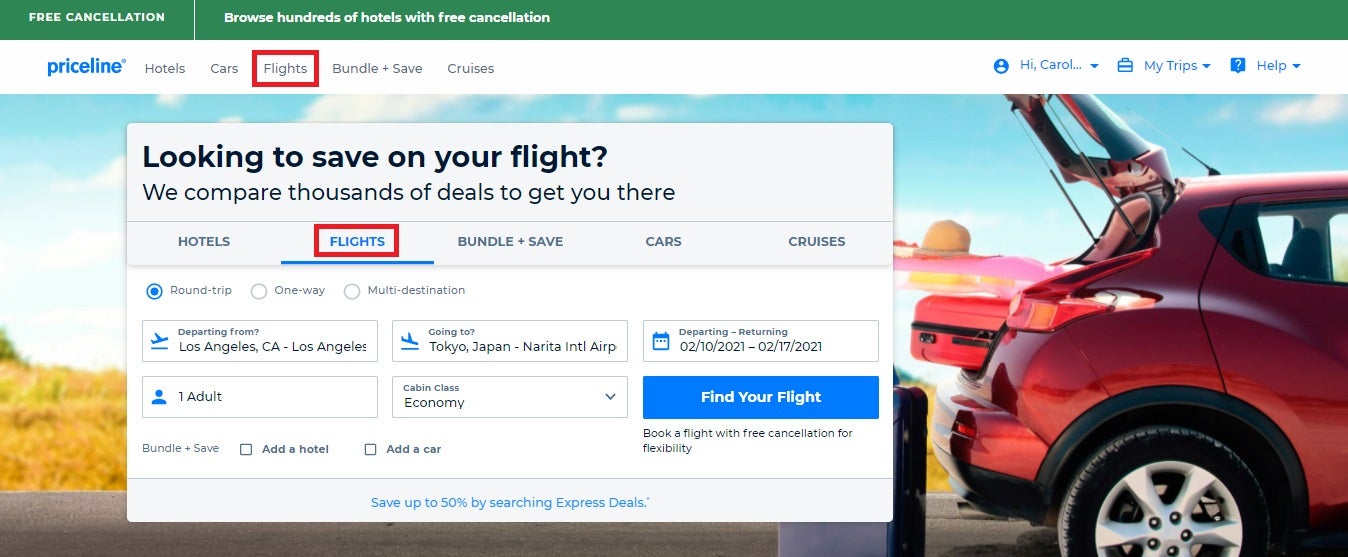The screenshot captures a Priceline desktop interface designed to assist with booking flights, hotels, cars, and more. The top section features a prominent, medium-green banner offering "Free cancellation" and "Browse hundreds of hotels with free cancellation." Below this banner, the Priceline logo appears in blue, accompanied by a horizontal menu bar with options in black text: Hotels, Cars, Flights (highlighted with a red rectangle), Bundle and Save, and Cruises. 

On the right-hand side, a user named Carol is greeted with a drop-down menu beside a torso icon. Additional options include "My Trips" with a suitcase icon, and a "Help" section symbolized by a blue and white question mark, both featuring drop-down menus.

In large black text, a headline advises: "Looking to save on your flight? We can pair thousands of deals to get you there." The user options below repeat the categories: Hotels, Flights (highlighted once again with a red rectangle and a blue underline), Bundle and Save, Cars, and Cruises. 

Flight booking options are presented in three bubbles: Round Trip (selected), One Way, and Multi-Destination. The departure location is "Los Angeles, CA, Los Angeles," and the destination is "Tokyo, Japan, Narita International Airport." 

The calendar indicates a departure date of February 10th, 2021, and a return date of February 17th, 2021. The trip is set for one adult in Economy class. There are additional options to add a hotel and a car under "Bundle and Save," though these are not currently selected.

A prominent blue rectangle button with white text prompts users to "Find Your Flight," highlighting the flexibility of booking with free cancellation. At the bottom, an offer to "Save up to 50% by searching Express Deals" is displayed.

The background image of the webpage depicts a travel scene in a rural area with a red car, one suitcase on the ground, and another in the car's trunk, symbolizing the travel and adventure spirit promoted by Priceline.

This descriptive caption thoroughly details the Priceline interface and guide for booking a flight.